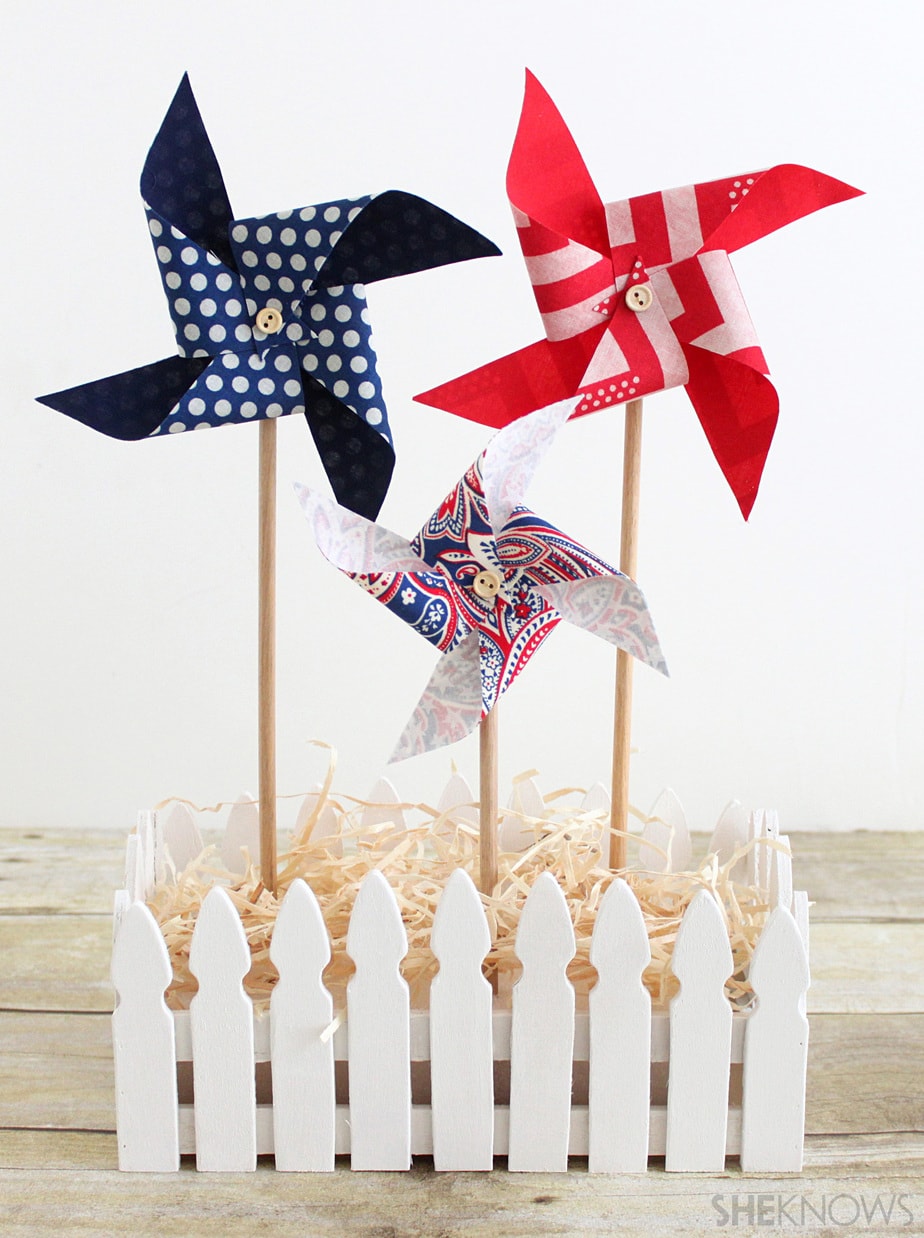This is a close-up photograph of a charming, patriotic-themed craft display. The base of the setup features whitewashed wooden planks, providing a rustic backdrop for the scene. At the center is a small, rectangular, white picket fence planter box filled with faux yellow hay. Standing upright in the hay are three festive pinwheels, each mounted on a wooden stick. The pinwheels showcase distinct designs: the left one is blue and white polka-dotted, the middle one boasts red and white stripes, and the right, shorter one has a red, white, and blue paisley pattern. Each pinwheel is adorned with a tan button at its center, adding a finishing touch to the whimsical display.